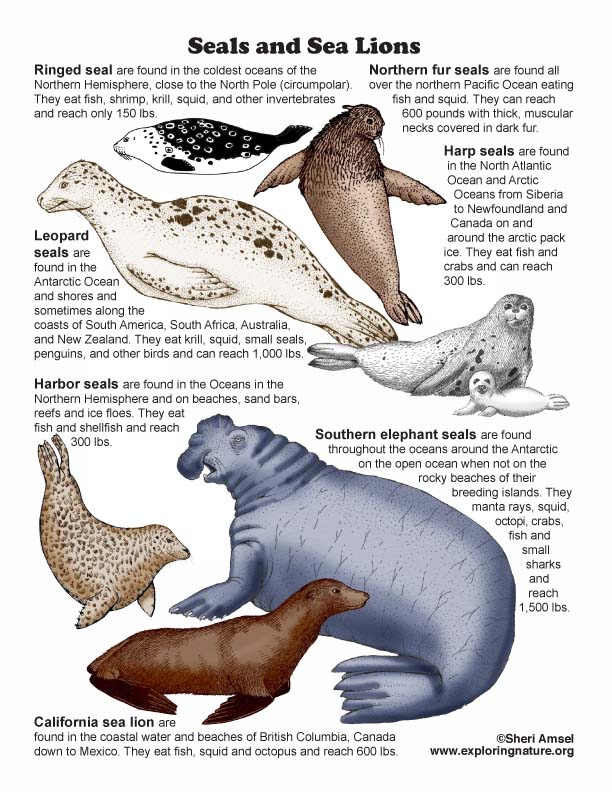This is a detailed color illustration focused on seals and sea lions, formatted in portrait orientation. At the top of the image, in bold black text, the title "Seals and Sea Lions" is prominently displayed. Directly beneath this heading, the illustration showcases multiple species including ringed seals, northern fur seals, harp seals, leopard seals, harbor seals, southern elephant seals, and California sea lions. Each animal is artfully depicted in various poses and orientations.

The top half of the image features four seals and sea lions with varied coloration and positions. The largest illustration, positioned at the bottom of this section, depicts a seal with brown spots on a cream-colored body, facing left. Above this, an illustration in black and white, also facing left, shows a seal with a black back and white spots. To the right of these, a vertically oriented light brown seal appears, while at the bottom right, a gray seal facing right looks back towards the viewer, accompanied by a baby.

In the bottom half of the illustration, three more seals and sea lions interweave their shapes, each species uniquely described by curved black text surrounding their forms. Detailed text around the image provides informative snippets about their habitats, diets (fish, shrimp, krill, squid, and other invertebrates), and physical characteristics, such as the ringed seals which are found in the coldest oceans of the Northern Hemisphere and reach only 150 pounds.

The illustrative style is a blend of color visuals and descriptive text, making this both an educational and visually appealing piece. At the very bottom right corner, the image credits the artist and source, "copyright Sherry Amayel Amzel, www.exploringnature.org," suggesting that it is likely part of a larger educational resource on a website.